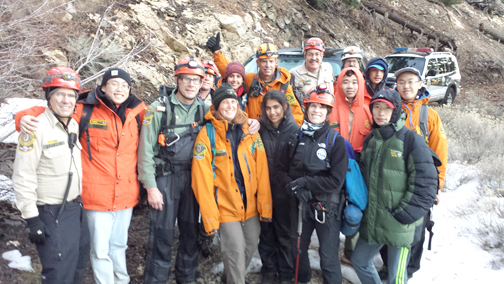In this color photograph, which is in landscape orientation, a diverse group of explorers is captured standing shoulder to shoulder on a snow-covered, mountainous road. They are warmly dressed in a variety of jackets, hats, and hoodies, indicative of the cold weather. There is no uniformity in their attire; some wear heavier outerwear while others sport lighter clothing that one might wear around the house. The group includes men and women of various ages.

Behind them, a police or sheriff's vehicle, easily identifiable by its red, white, and blue siren, is parked. Additionally, several vehicles belonging to the explorers are visible in the background. Among the group, a few individuals stand out, likely the guides, dressed in specific gear: two are wearing khaki-colored tops with black pants and red helmets, one in a green shirt with blue or gray overalls and a red helmet, and another in a yellow helmet with an orange jacket. The scene is set against a dirt bank with rocks and patches of snow, emphasizing the rugged, realistic nature of the environment. The explorers are looking up at the camera, smiling, creating an atmosphere of camaraderie and adventure.